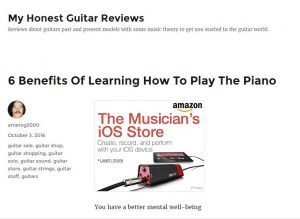A compact square screenshot primarily featuring a white background with black text overlay. At the top, the title "My Honest Guitar Reviews" is prominently displayed, followed by an illegible subheading. Below, the main heading "Six Benefits of Learning How to Play the Piano" stands out. On the left side, there's a small picture of a person with a mustache, accompanied by their screen name and the date "October 3rd, 2018." Beneath this, a short description is visible but too small to read clearly. To the right, there is a square image resembling an album cover. In the upper right corner, the word "Amazon" is mentioned. Below it, "Musician's iOS Store" is written in orange-ish font with the text "create, record, and perform with your iOS device" and a prompt to "learn more" underneath. The square image also includes what appears to be recording equipment. Below the entire layout, the phrase "You Have a Better Mental Wellbeing" is displayed.